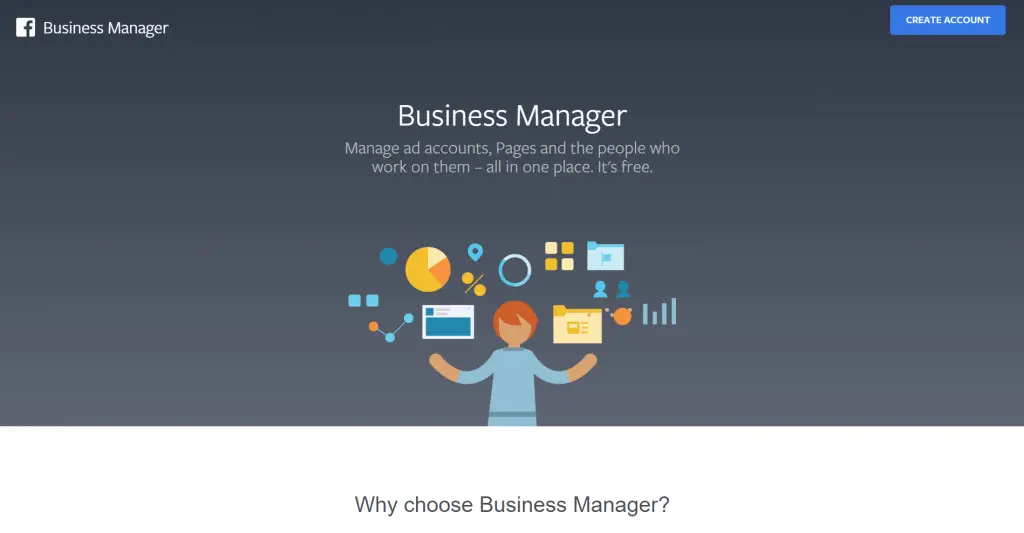This image depicts a webpage dedicated to Facebook's Business Manager. The header features the text "Business Manager" alongside the Facebook logo in white. Below the header, a blue "Create Account" button is prominently displayed, accompanied by the tagline: "Manage ad accounts, pages, and the people who work on them. All in one place. It's free." 

The main graphic on the page showcases an illustrated figure with red hair, dressed in a blue shirt and blue pants. Surrounding this figure are various icons, each floating above their raised arms. These icons include a yellow file folder, a blue bar graph, an orange and blue connected dots diagram, a pie chart, and a four-paneled yellow windows icon. Additionally, there are various pinpoints typically associated with enterprise software or applications dealing with numerical data.

Further down, the section titled "Why Choose Business Manager" stands out with a white background contrasting sharply against the gray backdrop of the rest of the page. The majority of the text here is white, with some black text near the bottom, providing additional information. Overall, the webpage appears designed to inform users about the benefits and features of using Facebook's Business Manager tool.